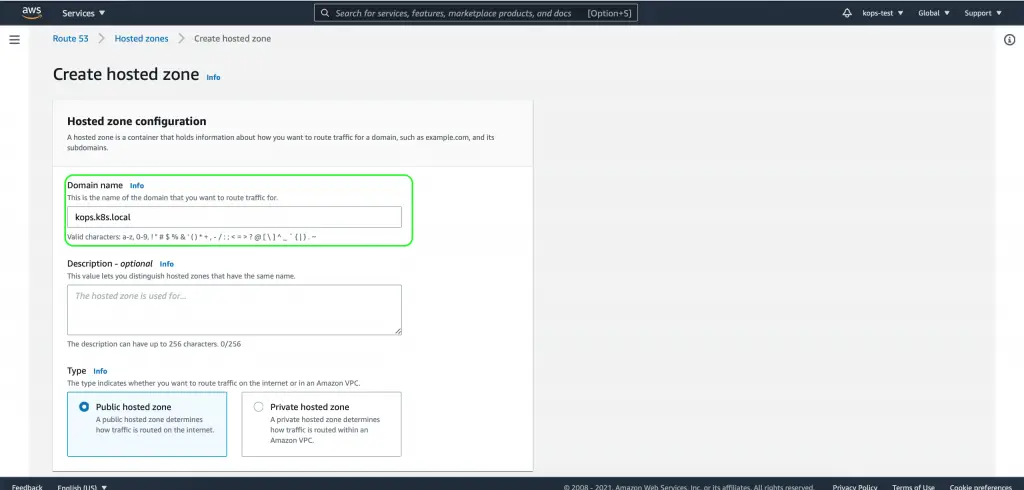The image depicts an administrative panel for AWS (Amazon Web Services). The interface features a black header spanning the top of the screen, containing the label "AWS services," a prominent search bar, a bell icon for notifications, global options, and support options. Directly below the black header, there is a white section that includes a hamburger menu.

Within the white area, the navigation highlights a path: Route 53 → Hosted Zones → Create Hosted Zone. The main heading below reads "Create Hosted Zone," with a subsection for "Hosted Zone Configuration." The configuration section describes a hosted zone as a container that holds information on how to route traffic for a domain, such as example.com and its subdomains.

A light green, curved-corner rectangle highlights the domain name entry area. Inside this section, there is a label for "Domain Name" followed by a blue link labeled "info," accompanied by an input field for the domain name entry. Below the input field, valid characters for the domain name are listed.

Further down, there is an optional "Description" field for distinguishing your hosted names within the panel. At the bottom of this configuration section, there are options for the type of hosted zone: "Public Hosted Zone" which is selected and outlined in blue, and "Private Hosted Zone," which is unselected.

The image cuts off at the bottom, revealing the presence of a black footer with text that is not legible.